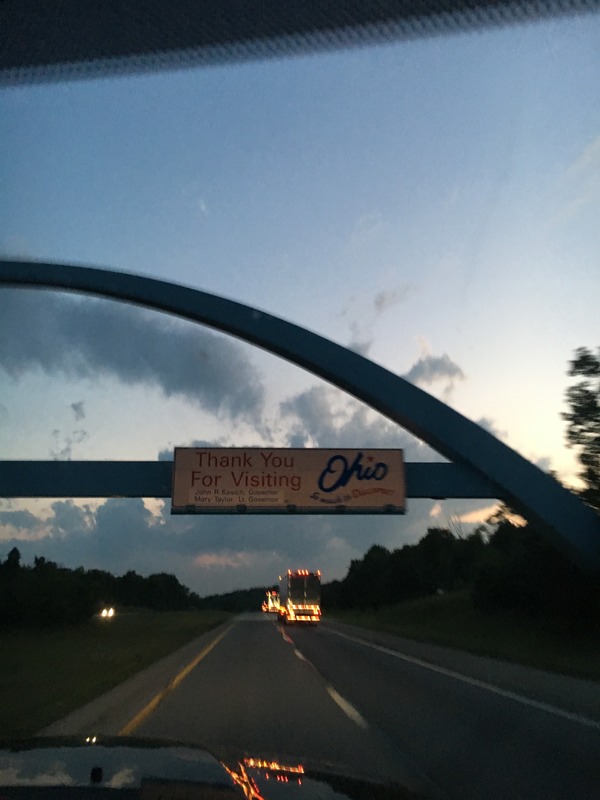The image captures a tall bridge spanning across a highway, prominently featuring a sign that reads "Thank you for visiting Ohio" in vivid red letters against a white background. The word "Ohio" is highlighted in blue, making it easily noticeable. The bridge stands elevated to provide clearance for large vehicles, including buses and trucks. Visible in the foreground are two large buses, with their rear lights illuminated, emphasizing the twilight setting as the sun descends. Surrounding the highway, lush trees frame the scene, and a car is in the process of passing under the bridge, accentuating the transitional moment as one leaves Ohio.